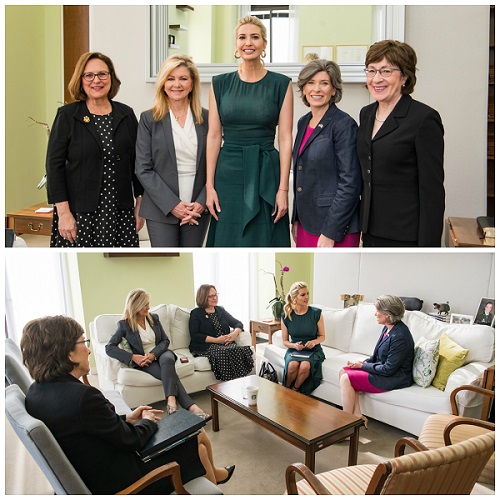This is a composite square image consisting of two photographs, one above the other, featuring the same five women. In the upper photograph, the group is standing in a row, all facing the camera. From left to right, the first woman has shoulder-length brown hair and wears glasses, a black and white polka dot dress, and a black jacket. The next woman has blonde shoulder-length hair and is dressed in a white top with a gray pantsuit. Positioned in the center is the tallest woman, identified as Ivanka Trump, who has her blonde hair pulled back and is wearing a sleeveless, long green dress. To her right, the fourth woman has salt-and-pepper hair and is attired in a blue blazer over a pink dress. The woman on the far right has short brown hair, wears glasses, and is clad in a black blazer. 

In the bottom photograph, the same women are seated in what appears to be a casual, parlor-like setting. They are positioned on a white loveseat, a couch, and two individual chairs, engaged in conversation. Various items such as notebooks and possibly a laptop suggest a business discussion. A brown table with a cup of coffee sits in the center, amidst additional unoccupied chairs. The surrounding environment features light lime green walls adorned with photographs and flowers, indicating a comfortable and informal atmosphere.